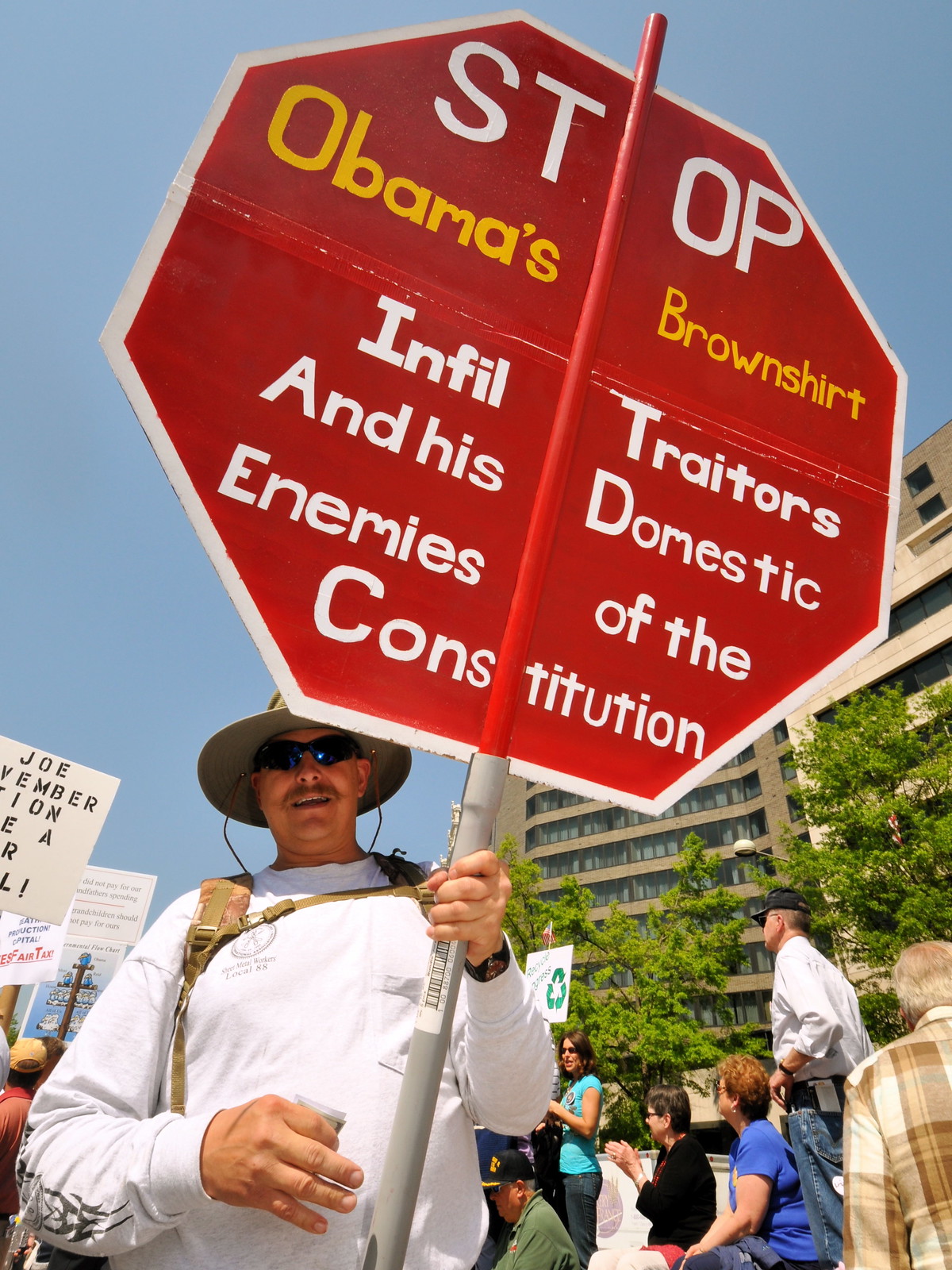In this photograph, a significant political protest scene is captured against the backdrop of clear blue skies, dominated by a demonstrator prominently situated in the foreground. This central figure, who is wearing a white long-sleeved shirt and a taupe-colored hat, stands out with a large homemade protest sign reminiscent of a traffic stop sign. The sign, attached to a gray pipe handle with a visible barcode sticker and a top half painted red, displays bold messaging in white and yellow letters. It articulates a strong opposition message: "Stop Obama's Brown Shirt, Infiltrators and His Domestic Enemies of the Constitution." Surrounding this main protester, a group of individuals are dispersed, some standing and others seated, all engaged in the peaceful protest. In the right background of the image, a tall, tan-colored high-rise building can be seen, enhancing the urban American setting, and suggesting that the protest took place some years ago given Barack Obama's tenure as President. Another visible protest sign in the distant background reads "Joe," presumably referencing Joe Biden, with partially obscured text likely related to an election in November. The overall scene offers a rich tapestry of political dissent, public assembly, and urban life.